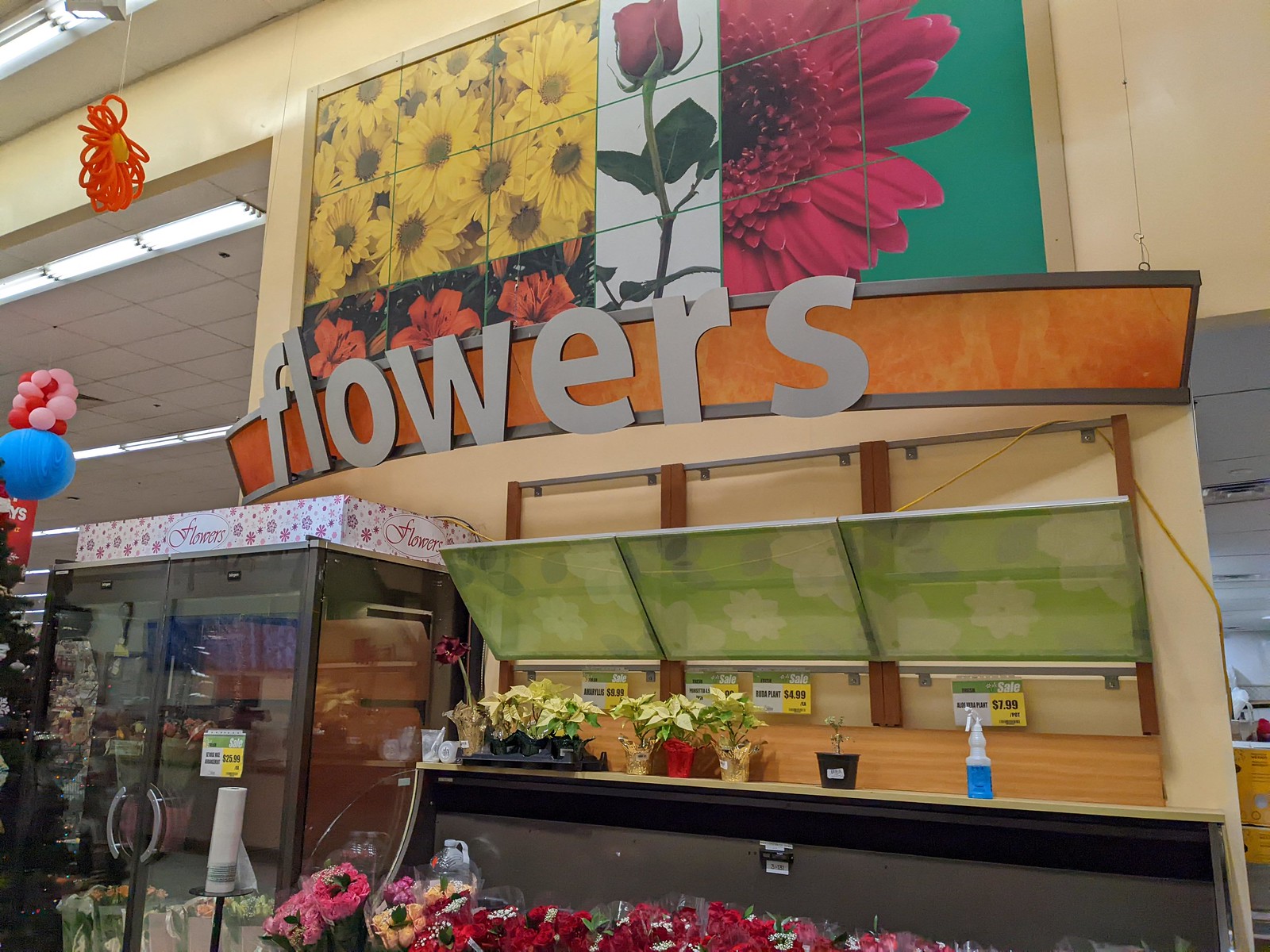This photograph captures the vibrant interior of a flower shop. At the top of the image, a large banner adorned with yellow sunflowers, orange blossoms, a rose, and a pink flower stretches across the scene. The banner sits on an orange backdrop, prominently displaying the word "FLOWERS" in bold white letters. Beneath the banner, a series of wooden wall mounts are decorated with green, silver, and white floral designs. Below these mounts, several sale price tags in shades of green, white, and yellow are visible. Flowers of various colors, including pink, red, burgundy, off-white, and pale yellow, rest on a ledge beneath the price tags, creating a lush visual display. To the side, a glass display case also features a green, white, and yellow price sticker, adding to the array of colorful and eye-catching details within the shop.